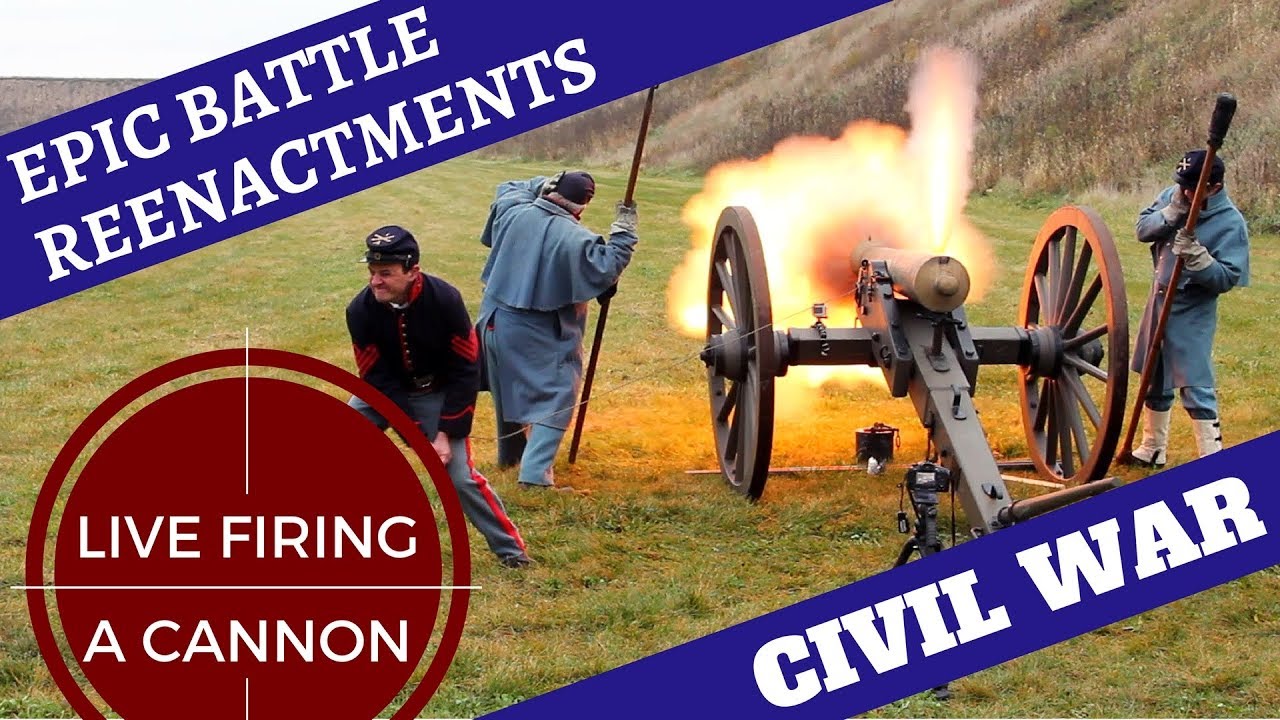The image is an advertisement for Civil War reenactments. In the upper left corner, on a blue background, white text diagonally reads, "Epic Battle Reenactments." Below this, there's a red circle with a crosshair, containing white text that says, "Live Firing a Cannon." In the lower right corner, another blue band features the words "Civil War" in white letters, emphasizing the historical significance with a nod to the phrase, "War is Hell." The photograph displays a grassy hill with three Civil War soldiers in Union uniforms operating a cannon. One soldier is pulling the firing string, while the other two are preparing the cannon, one facing away and the other checking the alignment. The cannon, mounted on two large wheels with a pivotal base, is poised for dramatic action.